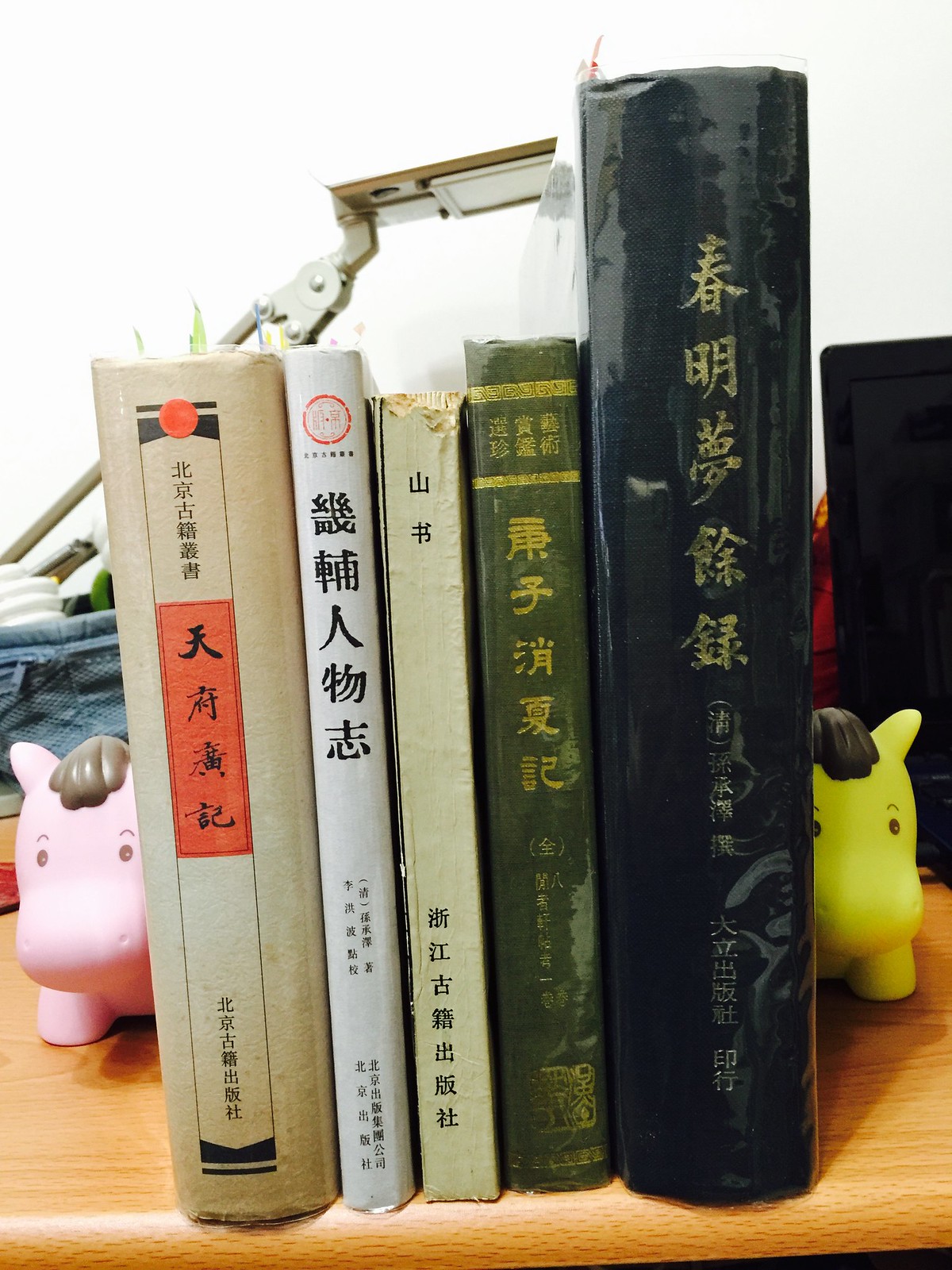In this photograph, a collection of books rests on a light brown wooden table characterized by some dark brown lines. The setup is flanked by two distinct horse-like figurines serving as bookends. The figurine on the left is pink with a small cluster of rounded hair, brown eyes that feature small white pupils, and round curved eyebrows. Beside it, there is a cloth bag that is blue, filled with various objects, and a brass-colored lamp with a flat, square-shaped top, currently turned off.

On the right side of the image, a yellow toy horse with brown eyes, white pupils, brown eyebrows, and brown hair peers partially obscured by the books. Additionally, a black laptop can be seen.

The books themselves are in what appears to be an East Asian script, possibly Japanese or Chinese. The collection features five main books: Starting from the left, there is a tan book with an orange sun at the top of its spine, followed by a white book with an orange logo. In the center is a light green tattered book with parts ripped, followed by a dark green book adorned with gold embroidery and letters. Finally, a tall, glossy black book with gold writing oriented from top to bottom is situated on the far right. This arrangement is set against a white wall.